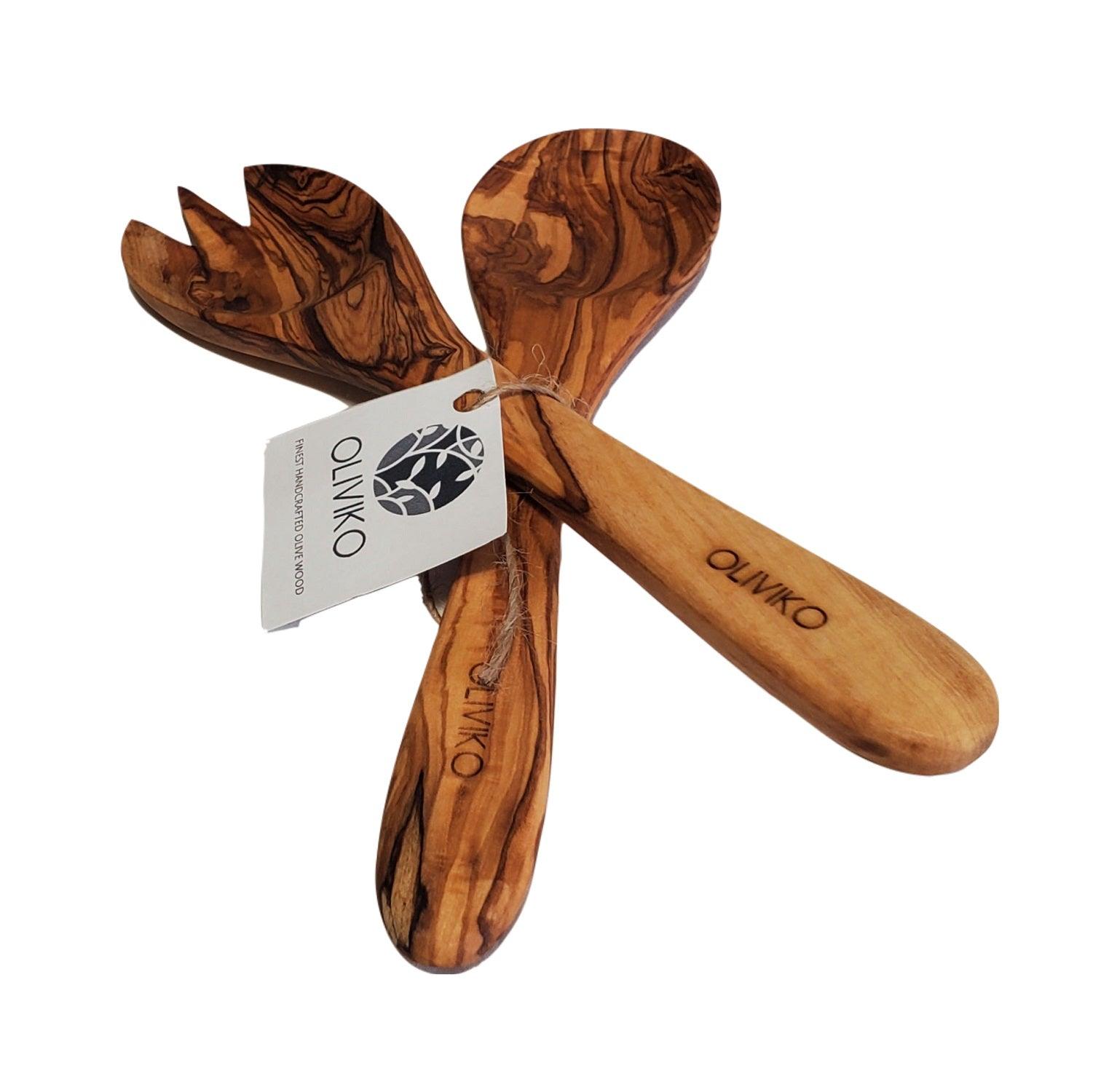The image depicts a pair of wooden serving utensils against a plain white background, showcased prominently in the center. The set consists of a large spoon and a large fork designed for tossing salads, featuring rich brown marbling that gives each utensil a unique wood grain texture. The utensils are made of a darker-hued olive wood, exuding a high-quality craftsmanship. They lie crisscrossed over each other, bound together with twine that secures a white rectangular tag. This tag has a circular logo displaying white vines and leaves on a black background, and the brand name "Olivico" elegantly written beneath it in black text. Additional text on the tag reads "finest handcrafted olive wood." Engraved on the handles of both the spoon and fork is the word "Olivico," highlighting the artisanal quality of the product.